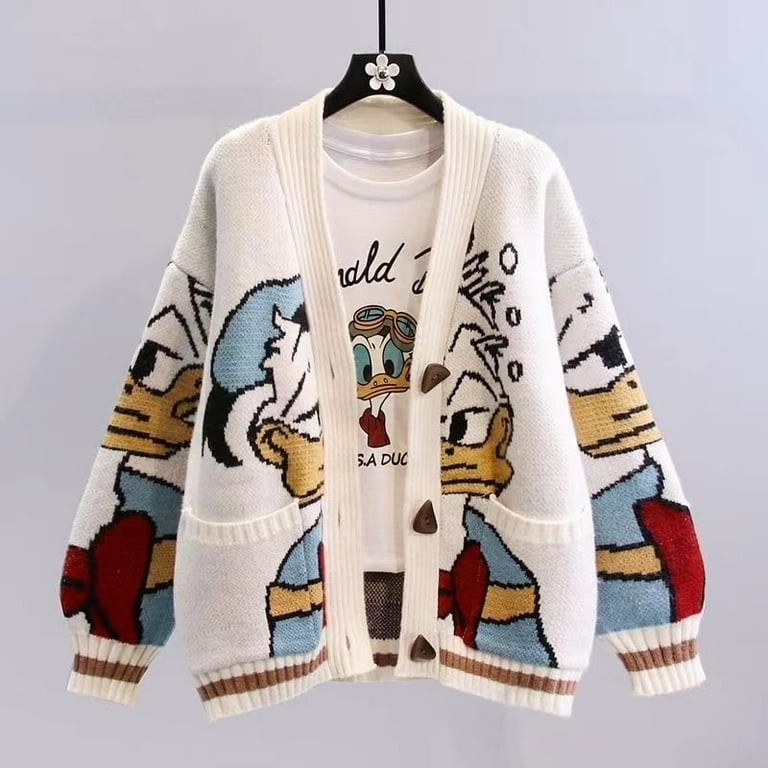This color photograph features a black hanger adorned with a white flower, set against a soft light gray background. The hanger holds a white cardigan sweater, which is open and visibly unbuttoned, revealing a white T-shirt behind it. Both the cardigan and the T-shirt prominently feature intricate designs of Donald Duck. The cardigan's design spans its full sleeves and center, showing parts of Donald Duck's face divided by the button seam. Donald Duck is illustrated wearing a blue hat, a blue and yellow sweater, and his iconic red scarf. The edges and bottom sleeve ribbing of the cardigan display a distinct pattern with alternating white and brown stripes. The T-shirt beneath the cardigan also showcases Donald Duck, complete with blue eyes, a yellow beak, and goggles on his head, though much of it is obscured by the cardigan. The overall composition creates a whimsical yet cohesive portrayal of the beloved Disney character.